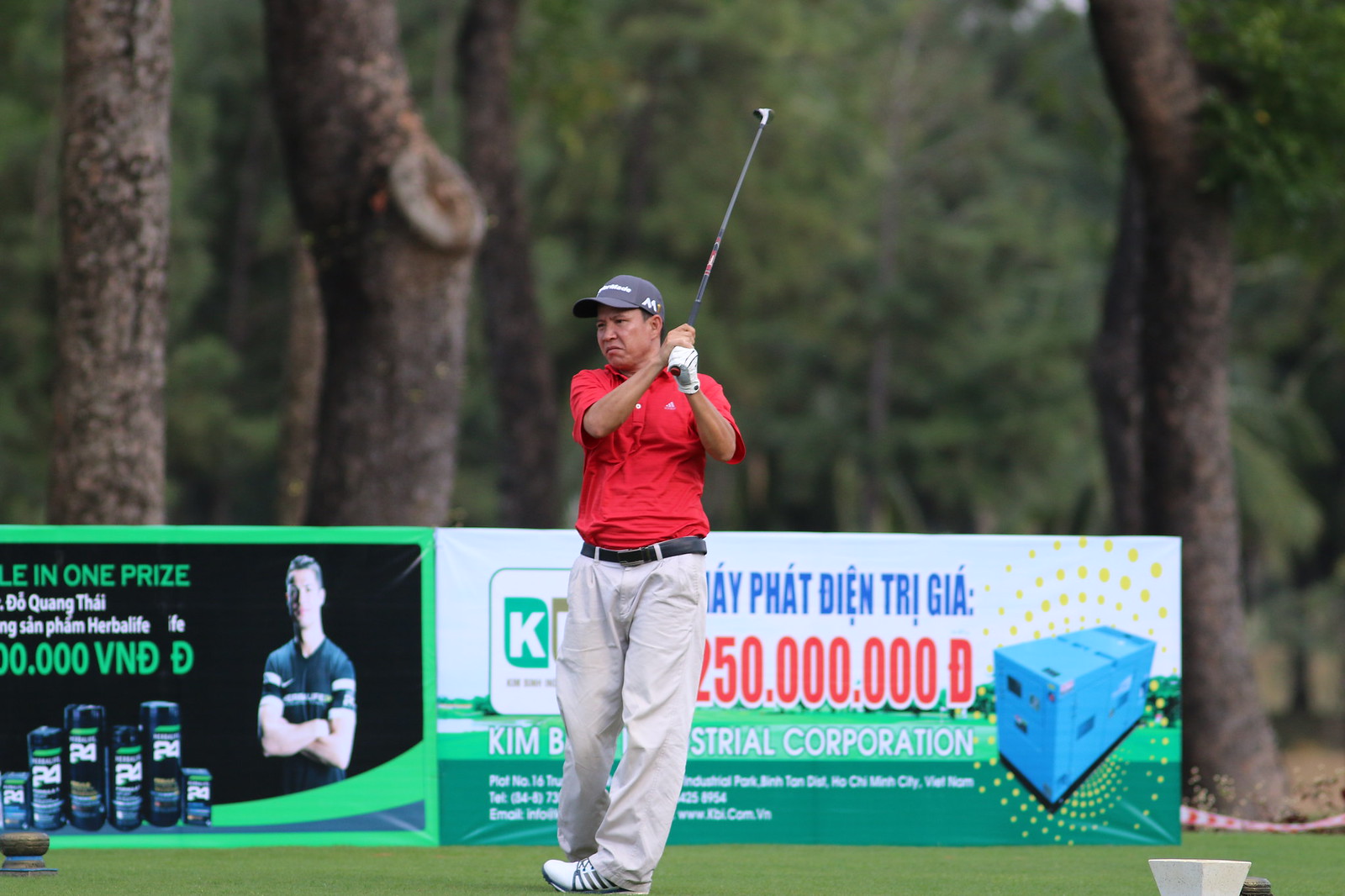In an outdoor scene on a golf course, a man stands tall, seemingly having just completed a swing. He wears a bright red polo shirt, khaki pants, a black belt, and white and black cleated shoes. A gray cap shades his eyes as he holds his mostly black golf club with red accents and white stripes aloft. His left hand is gloved, and he has a somewhat sour expression on his face. The backdrop features a forest area with younger pine trees. Behind him, a large, mostly green sign with red print advertises various products, potentially protein powder or body sprays, and includes a prominent red number—250 million D. To his right, a banner in another language promotes a big, blue, rectangular item, adding to the commercial ambiance of the setting.